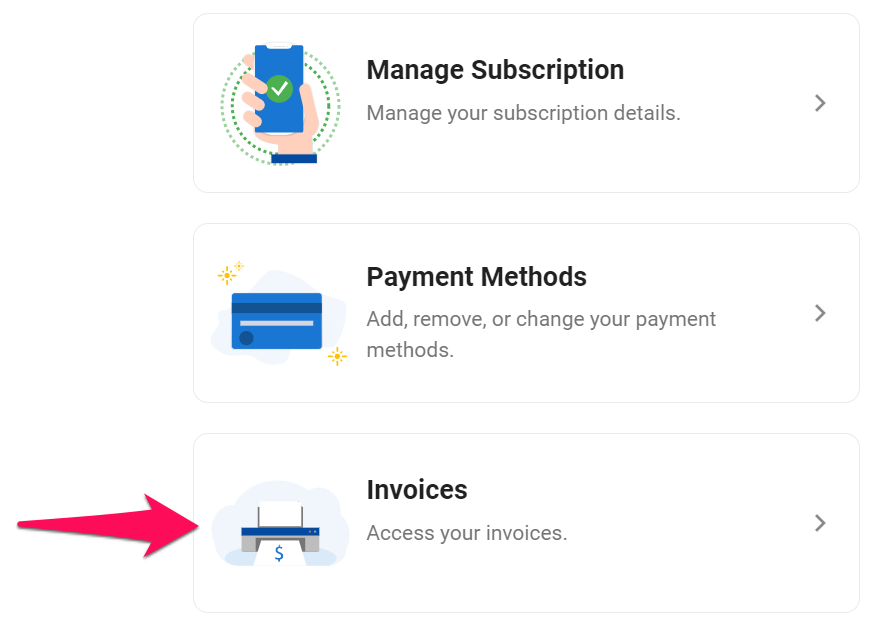The image appears to be a screenshot from a website's subscription management page. The interface is set against a white background and features three rectangular sections with rounded corners outlined by a thin grey line.

1. **Manage Subscription**: The top section has the title "Manage Subscription" in black text, accompanied by the subtitle "Manage your subscription details." On the right side, there is a small arrow indicating more options. The left side features an illustration of a hand holding a blue phone with a green checkmark displayed on its screen. The hand has a blue sleeve, and the phone is encircled by two coils of green wire.

2. **Payment Methods**: The middle section is labeled "Payment Methods" with the description "Add, remove or change your payment methods" beneath it. A right-facing arrow is on the right, similar to the first section. The left side shows an infographic of a credit card, specifically the back view. The card is blue with a series of colored stripes: a black stripe at the top, a white stripe below it, and a dark blue stripe further down. It also features a blue circle and yellow stars positioned at the top left and bottom right.

3. **Invoices**: The bottom section is titled "Invoices" with the guide "Access your invoices" below the header. Another arrow points to the right for further navigation. To the left, there is an image of a grey printer with a blue top, ejecting a page marked with a blue dollar sign. A light blue background highlights the printer. Additionally, a red arrow extends from beyond the left side of this section, pointing towards the printer illustration, becoming wider towards its right end.

This detailed caption thoroughly describes the layout and visual elements of the website's subscription management interface.